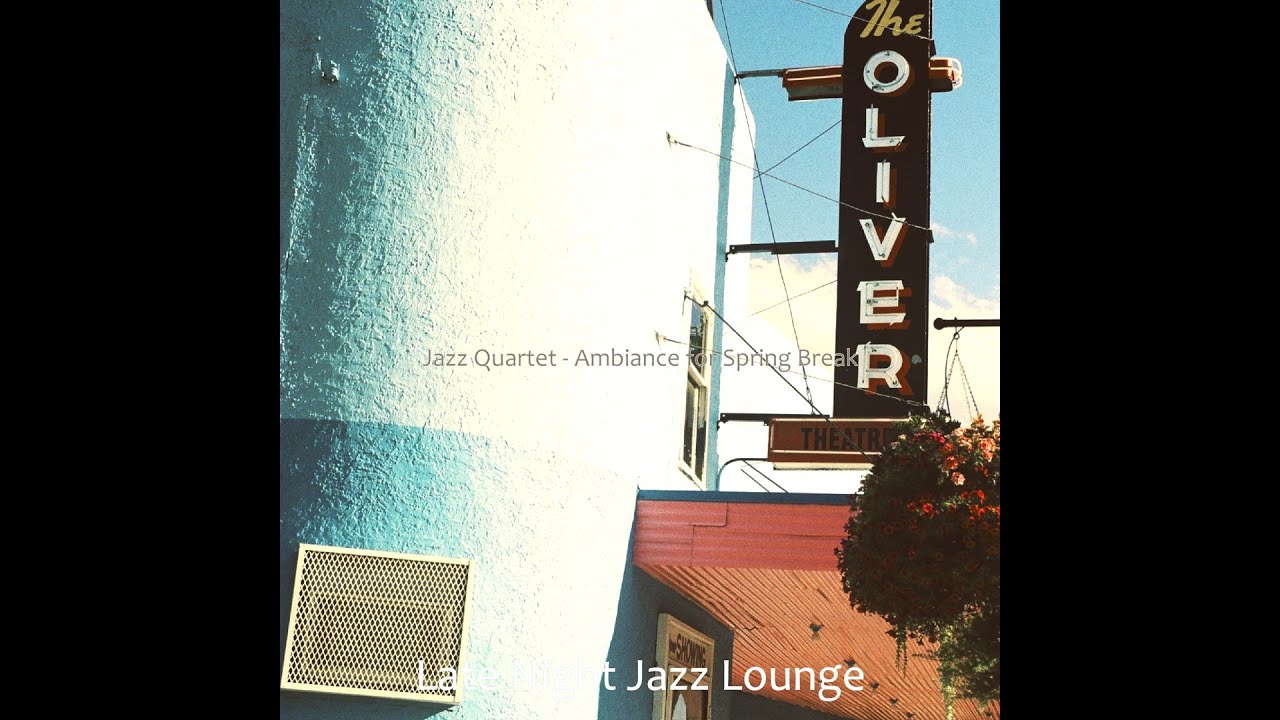This detailed photographic image captures the exterior of "The Oliver," a jazz lounge, set in an outdoor scene under a clear blue sky with visible support wires. The white stucco building has a distinct curved corner and features a mix of modern and vintage elements. Prominently displayed on the right side of the building is a black-mounted sign with "The" on top and "Oliver" spelled vertically, suggesting possible neon lighting for nighttime illumination. Below the sign is a black or dark brown rectangle reading "Theater" at the bottom, indicating the venue's full name: "The Oliver Theater."

High up on the building's facade, there is a wood canopy over the front door, adorned with a couple of hanging baskets on the right side. A vent is noticeable in the lower left-hand corner, and an outdoor speaker is mounted nearby, hinting at the lively ambiance within. The lower right corner features the building’s awning, with visible greenery enhancing the scene.

Text overlays add context: "Late Night Jazz Lounge" is written in white at the bottom, while "Jazz Quartet-Ambience of Spring Break" appears in small gray letters across the center, subtly branding the jazz club's seasonal theme. Black vertical borders frame the left and right sides of the image, lending a distinctive, inset appearance to the central square photograph.